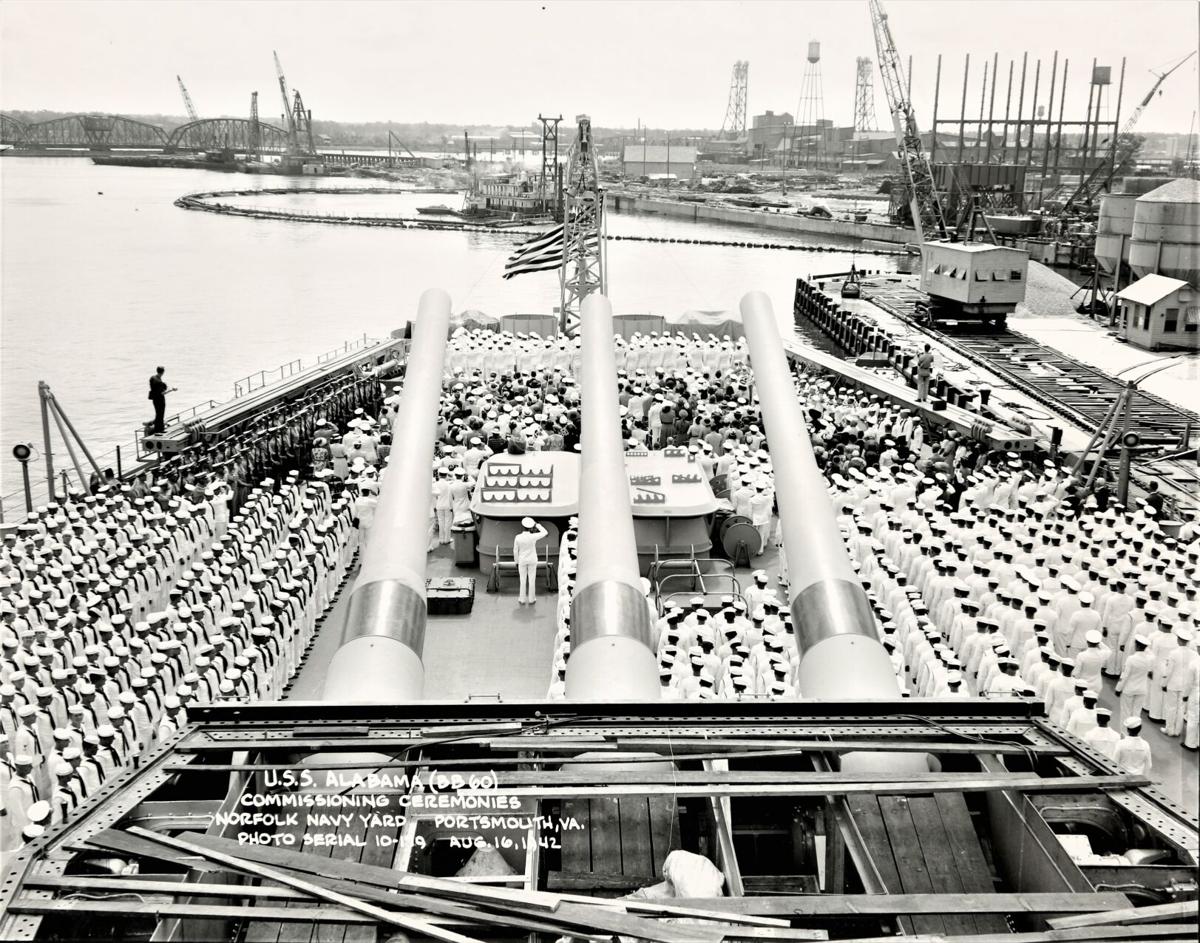This is a black-and-white photograph capturing the commissioning ceremony of the USS Alabama (BB-60) at the Norfolk Navy Yard in Portsmouth, Virginia, on August 16, 1942. The image is taken from a high vantage point, offering a top-down perspective of the battleship. Dominating the scene are three prominent white cannons extending outward from the ship's deck. Rows of naval sailors, all dressed in white uniforms and hats, stand in neat formation facing away from the camera, their backs visible. Some are saluting, reinforcing the ceremonial tone. Beyond the ship, the scene reveals a large body of water, with various landmarks such as a bridge in the upper left, buildings, and land on the right. Noteworthy details include a cable car, oil drums, a little building, and a large ladder structure emerging from one of the buildings. The words "USS Alabama Commissioning Ceremonies Norfolk Navy Yard, Portsmouth, Virginia" are inscribed in white font at the bottom left of the photograph, alongside the serial number "Photo Serial 10-19."